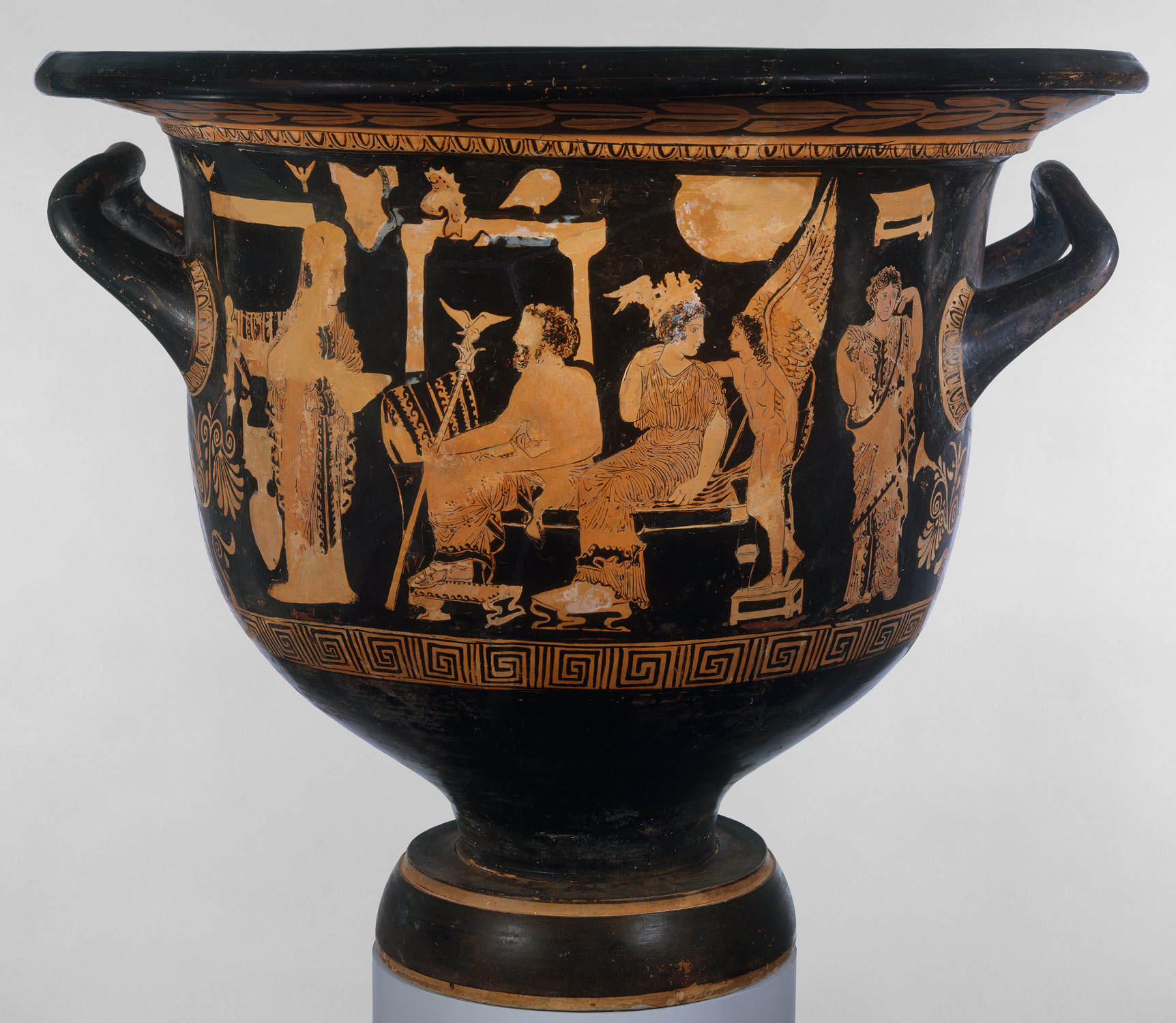This is a detailed square image featuring an ancient Grecian urn against a light gray background. The urn, predominantly black and shiny, suggests it has been fired in a kiln. Its base is ornate, with a combination of dark brown and gold trims, possibly on top of a round, light blue stand. The urn features two black handles on either side, extending to a narrow base and culminating in a dark brown rim with a possible leaf-like gold pattern.

The urn is adorned with intricate, etched scenes and patterns in shades of orange, tan, brown, rusty gold, and white. The central artistic scene on the urn’s body depicts several Grecian figures in a rusty brownish gold color, each in classical attire with notable details. Starting from the left, there is a priest-like figure, although chipped, holding a vessel. Next, a man sits on a couch with a robe draped over his legs, holding a staff topped with an eagle. Beside him, a woman in a toga with an ornate crown, seemingly featuring Pegasus horses, looks toward an angelic figure with feathered wings, standing on a stool to meet her gaze. Lastly, another figure in a robe stands with hands raised in a "woe is me" gesture.

The urn features a spiral maze-like pattern at the bottom, and both the top and bottom regions are decorated with abstract gold designs – described as thick coils at the bottom and neat rows of gold nail or tooth-like patterns at the top. The detailed craftsmanship and the colors employed give the urn a highly ornamental and ancient appearance.